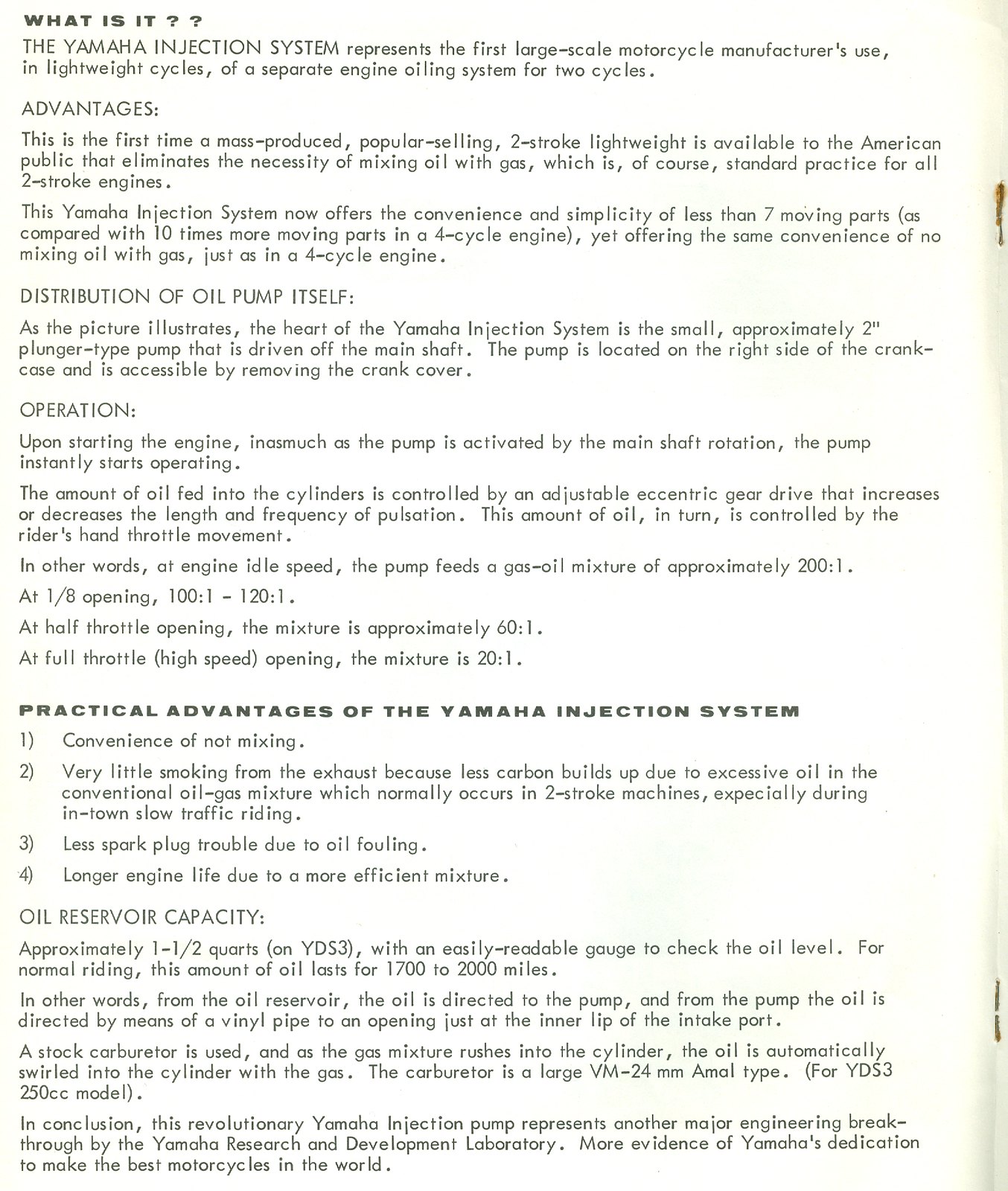This image captures a detailed page from a Yamaha instruction manual, highlighting the groundbreaking Yamaha injection system. The document, black and white on white paper, features a header that reads, "What is it?" Following this, it elaborates on the Yamaha injection system being the first major use of a separate engine oiling system in lightweight two-cycle motorcycles by a large-scale manufacturer. The page outlines the numerous advantages of the system, such as eliminating the need to mix oil with gasoline—a common requirement for two-stroke engines. This feature parallels the convenience of four-stroke engines, which typically do not require this mixing.

It details the system’s mechanics, including the oil distribution pump, a small plunger-type device driven by the main shaft and located on the right side of the crankcase. This pump starts working as soon as the engine does, adjusting the oil-to-gas ratio based on throttle position: idle (200:1), one-eighth open (100-120:1), half-throttle (60:1), to full throttle (20:1). Practical advantages listed include reduced exhaust smoke, fewer spark plug issues due to oil fouling, and extended engine life thanks to more efficient oil mixing. The document also notes that the oil reservoir, with a capacity of approximately 1.5 quarts, can support normal riding for 1,700 to 2,000 miles. It explains that the oil is pumped through a vinyl pipe and mixed with the gasoline as it enters the cylinder, facilitated by a stock carburetor—a VM 24-millimeter Amal type on the YDS3 250cc model. In conclusion, the manual emphasizes the Yamaha injection pump as a significant engineering achievement by Yamaha, aimed at enhancing the performance and convenience of their motorcycles.